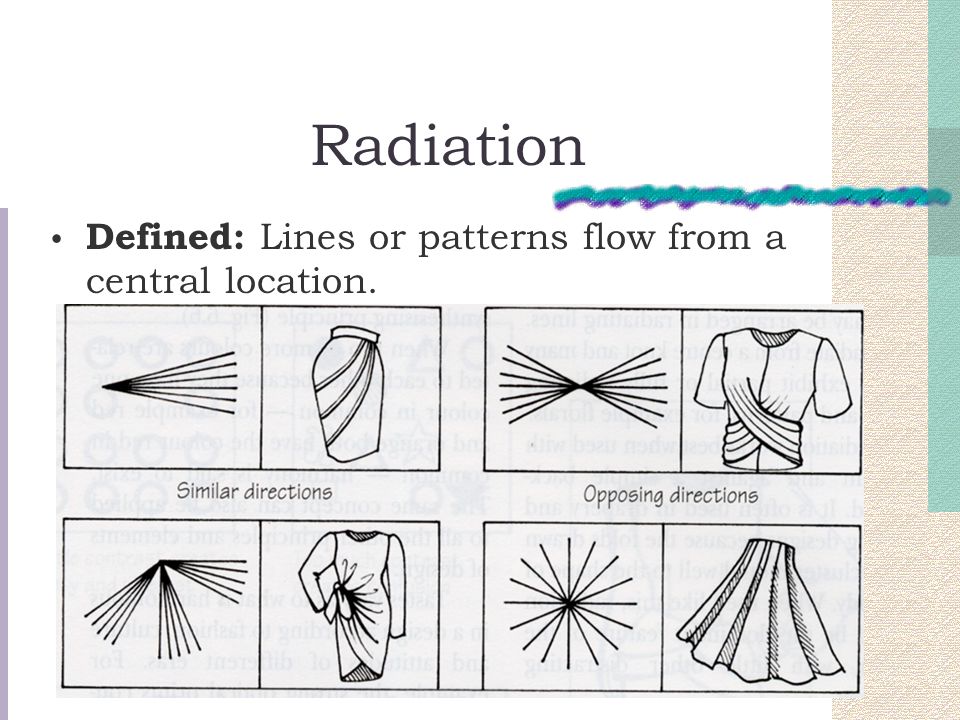The image appears to be a detailed informational graphic, possibly from a PowerPoint presentation, focused on the concept of radiation in the context of art and fashion design. The background is predominantly white, with a strip of teal and tan colors along the right side, enhancing visual appeal. At the top center, the word "Radiation" is prominently displayed in bold black font, immediately followed by the term "Defined:;" which introduces the definition: "Lines or patterns that flow from a central location."

Below the text, the graphic features four pairs of boxes. Each pair consists of a left box showing hand-drawn lines illustrating the radiation pattern, and a corresponding right box depicting a hand-drawn example of this pattern applied to women's clothing items, such as skirts and dresses. The left-most four boxes are labeled "Similar Directions," demonstrating how lines or pleats flow in the same direction, while the four boxes on the right are labeled "Opposing Directions," showing patterns where lines flow in opposite directions.

For example, one set includes a star-shaped radiation pattern, juxtaposed with a drawing of a black and white skirt featuring similar directional pleats. All illustrations are hand-drawn, contributing to the instructional and artistic quality of the graphic. The image effectively uses color and illustrative examples to clarify the artistic concept of radiation, distinct from its scientific connotation.